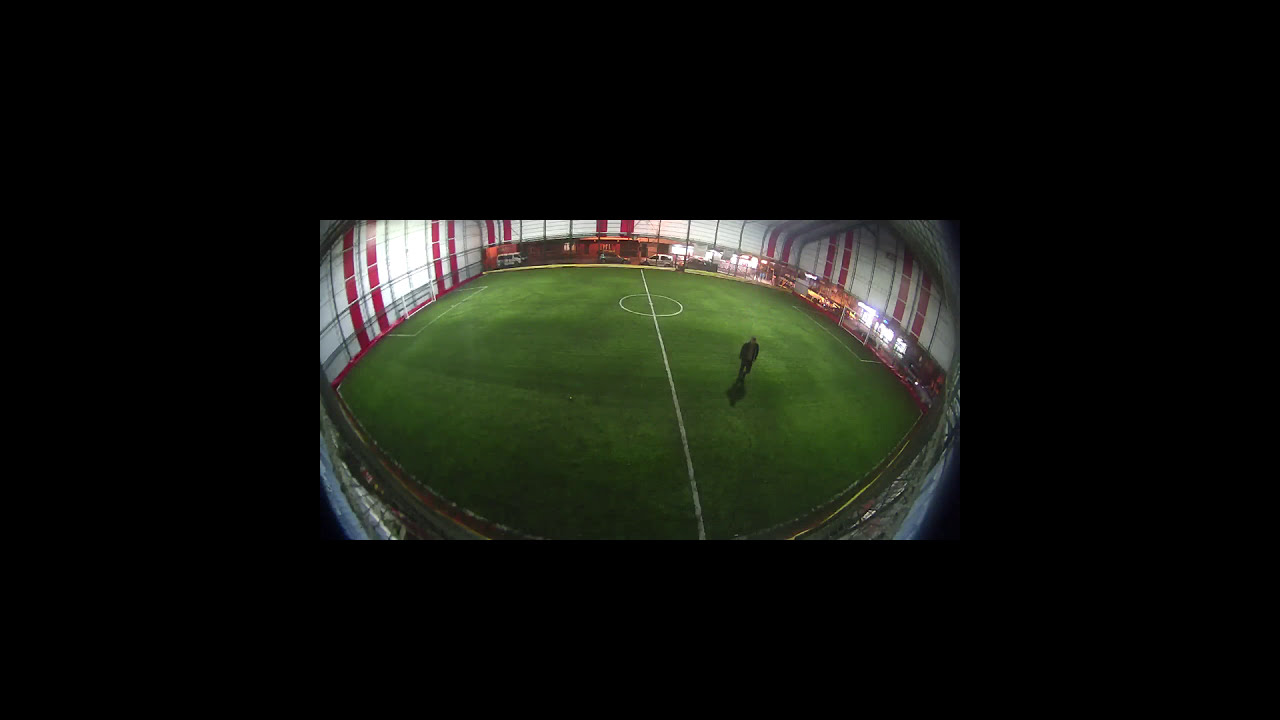The image depicts an indoor soccer arena with lush green turf that varies slightly in shade. A central white line bisects the field, complete with a circle in the middle. The arena is circular in shape and features white walls accented with intermittent red vertical stripes. Surrounding the perimeter is a fencing-like structure. Captured from above with a fisheye lens, the image gives a wide, somewhat distorted view, resembling a security camera's perspective. A man dressed in black stands alone on the field. Outside the arena, visible through the curved roof, there's a brown building with cars parked in front, suggesting recent or upcoming activity. The image itself is quite small and is encased in a large black border that makes some additional features, like potential scaffolding or pipes, difficult to discern.